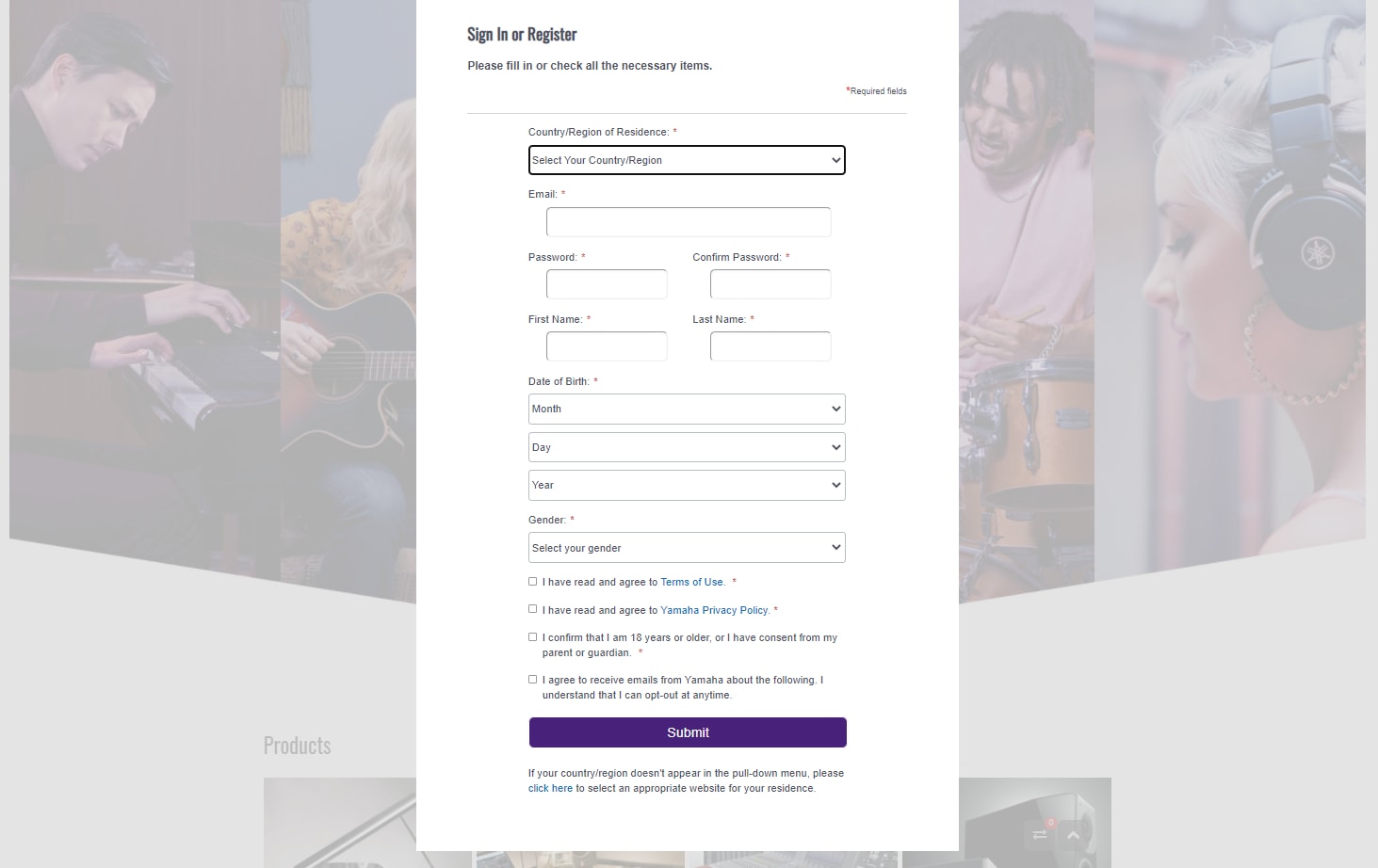The image displays a sign-in or registration page for Yamaha, the renowned musical instrument manufacturer. In the background, a diverse group of musicians is engaged in their craft: 

- A man with black hair, dressed in a black long-sleeve shirt or turtleneck, is passionately playing the piano.
- A blonde-haired woman is strumming a guitar with focus and dedication.
- Another man, sporting stylish dreadlocks and dressed in a pink shirt, is energetically playing the drums.
- There is also a blonde-haired woman wearing large hoop earrings and headphones. Her role is ambiguous, but she might be singing.

In the foreground, the sign-in or registration form is prominently displayed. The form is primarily white with black text and includes fields for "Country/Region of Residence," "Email," "Password," "Confirm Password," "First Name," "Last Name," and "Date of Birth" (specified by month, day, and year). Users are prompted to select their gender and tick several acknowledgment boxes:

1. "I have read and agreed to the terms of use."
2. "I have read and agreed to the Yamaha privacy policy."
3. "I confirm that I am 18 years or older and I have consent from my parent or guardian."

Additionally, there is an optional checkbox for agreeing to receive promotional emails from Yamaha, with an understanding that users can opt out at any time.

Compulsory fields are marked with red asterisks, ensuring users complete them before proceeding. At the bottom of the form is a prominent purple "Submit" button with the text in white, inviting users to finalize their registration.